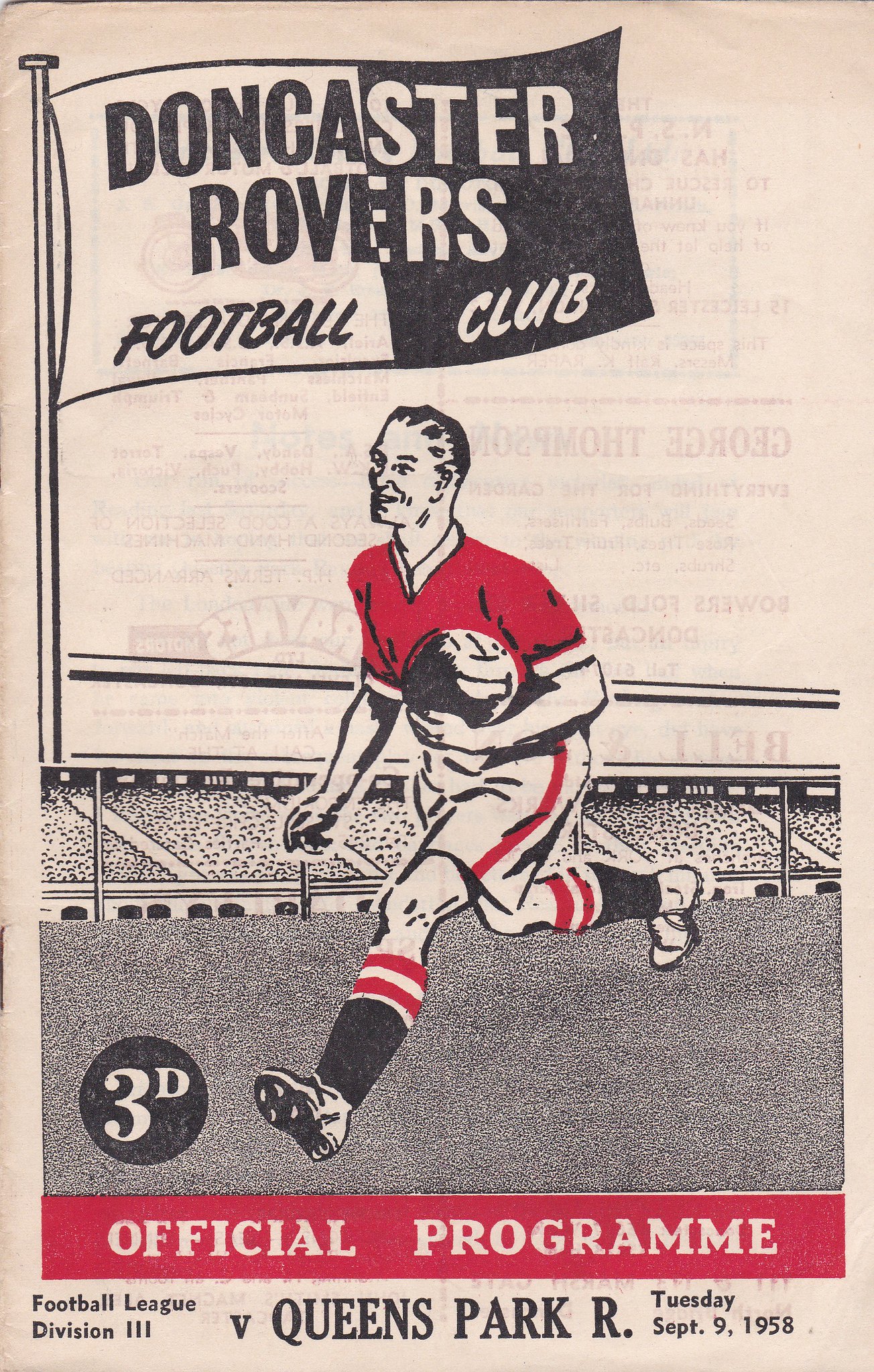This image depicts a vintage-style poster for the Doncaster Rovers Football Club, prominently featuring a cartoonish illustration of a man carrying a ball, which looks like it could be a soccer ball or a volleyball. The man is depicted in a red shirt and white shorts with red stripes, complemented by classic white socks with red stripes around the calves. He also wears black socks with white and red stripes at the top. Above the man, an illustrated flag with a unique design—half black and half white—waves proudly, with the text "Doncaster Rovers Football Club" cleverly written in contrasting colors to match the flag's background.

To the bottom left of the poster, there's a black circle showcasing a large number '3' and a small 'd'. Below this detail, a red-bordered section with a red background announces "Official Program, Football League Division III, V Queens Park, R, Tuesday, September 9th, 1958." The program spelling reflects the traditional British format with two M’s and an E. Although a drawing rather than a photograph, the man is depicted on what appears to be a football field, capturing the essence of the sport and the era.